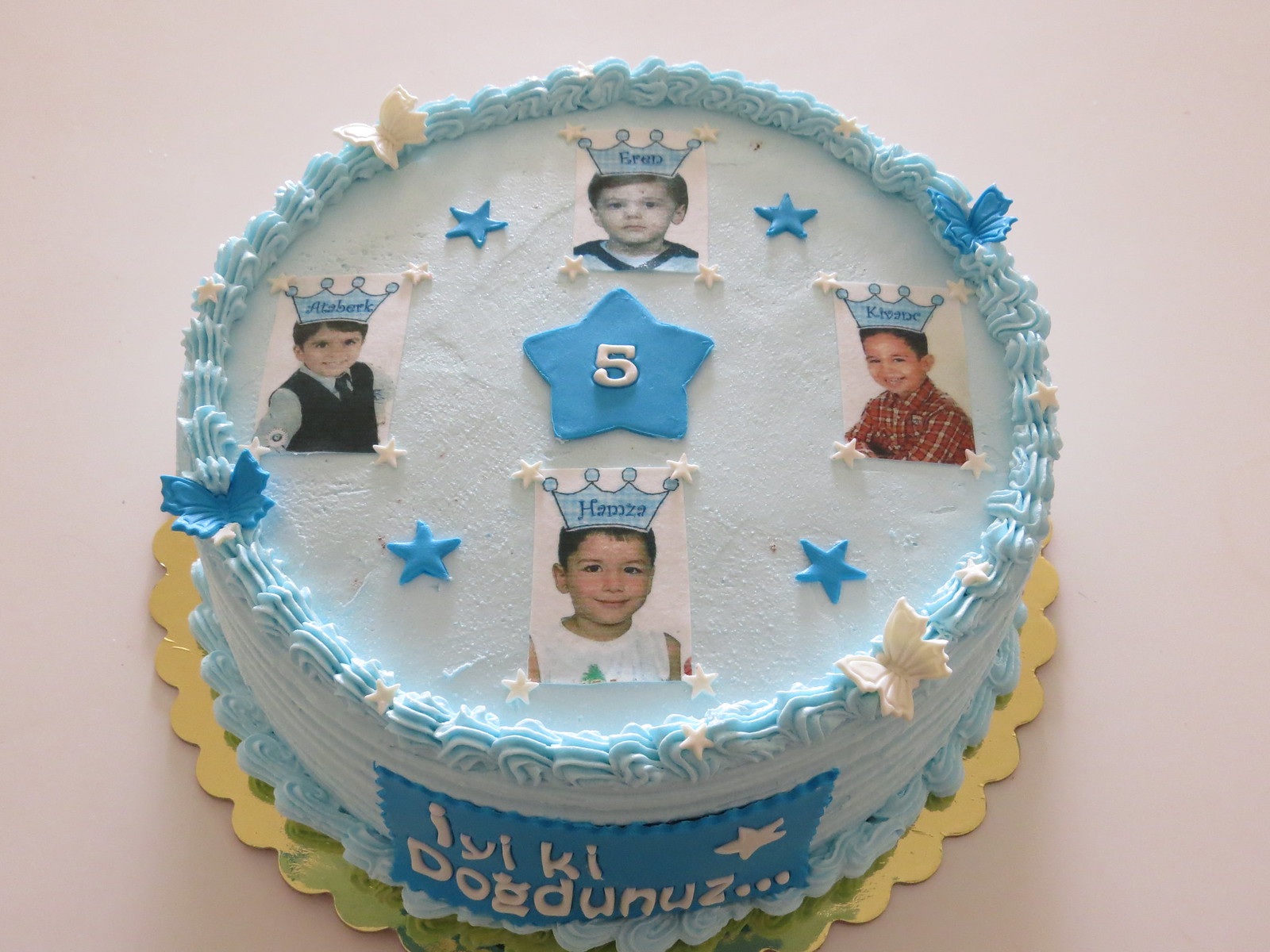This is an indoor digital photograph of a birthday cake resting on a golden plate against an off-white to pinkish background. The cake is predominantly blue with intricate white icing forming a border around the top. The surface of the cake features four well-decorated white and blue butterflies positioned at the bottom right, left-hand side, top upper portion, and coming around to the right. At the center of the cake, there is a prominent blue star with a white number 5, symbolizing the age being celebrated.

Surrounding this central star, the top of the cake displays four pictures of a young boy adorned with a blue crown, each positioned at the top, bottom, left, and right sides of the cake. Blue stars are sprinkled across the surface of the cake, adding to the celebratory design.

A blue rectangular plaque with the writing "IYIKIDOGDUNUZ"—suspected to be a celebratory message in another language—is attached to the front of the cake. The cake conveys a festive birthday atmosphere as it honors the young boy’s fifth birthday with meticulously detailed decorations.